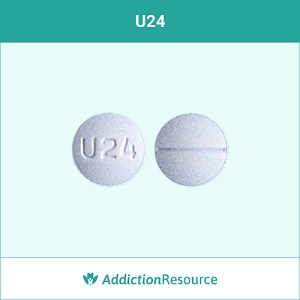The image features a teal-colored rectangular banner at the top that spans the entire width from left to right. Within this banner, there is white text in capital letters that reads "U 24." Below the teal banner, the background shifts to a light green color, covering the majority of the remaining area. Centrally positioned in this light green section is a detailed depiction of a pill, showing both its front and back views. The pill appears light gray, though it might be intended to look white. On the front view, the left side of the pill is marked with the text "U 24" in capital letters. The back view of the pill features a single horizontal line running across it. The bottom of the image contains a white rectangular box. On the left side of this box, there is an unidentified icon. On the right side, the text "Addiction Resource" is written in light green font, with "Addiction" in italics and "Resource" in regular type.